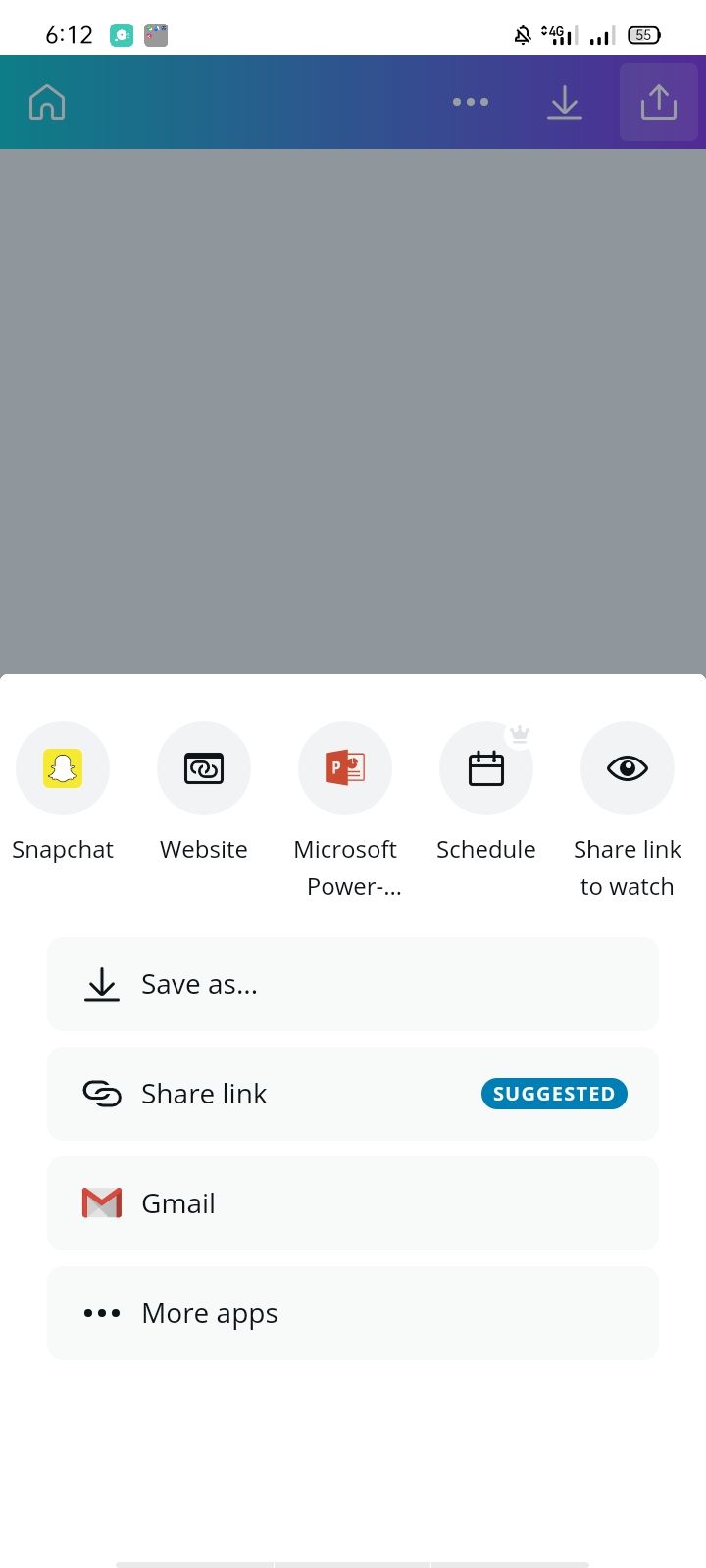This is a detailed screenshot from a mobile phone interface:

- **Top of the Screen:** 
  - A white status bar with dark gray font indicating the time as 6:12.
  - Two gray square icons.
  - A bell icon, indicating notifications.
  - A 5G symbol with three out of four signal bars.
  - A 4G signal indicator also showing three out of four bars.

- **Below the Status Bar:**
  - A purple bar featuring a "Home" icon on the left and a "Download" icon on the right.

- **Below the Purple Bar:**
  - An empty gray box.

- **Below the Gray Box:**
  - A white bar with multiple small icons/apps:
    - Snapchat icon.
    - An icon labeled "Website."
    - Microsoft PowerPoint icon.
    - A calendar icon labeled "Schedule."
    - An eye icon with a label that reads "Share link to watch."

- **Below the Icon Bar:**
  - An off-white rectangle with black text that says "Save As."
  - Another off-white rectangle that says "Share Link."
    - At the right end of this rectangle is a blue oval with white text that reads "Suggested."

- **Below the "Share Link" Rectangle:**
  - A rectangle labeled "Gmail" with the Gmail icon (an envelope with an "M" on it).

- **Bottom of the Interface:**
  - Another bar that reads "More Apps."

Each element provides a clear and organized overview of the phone's notification and app management system.